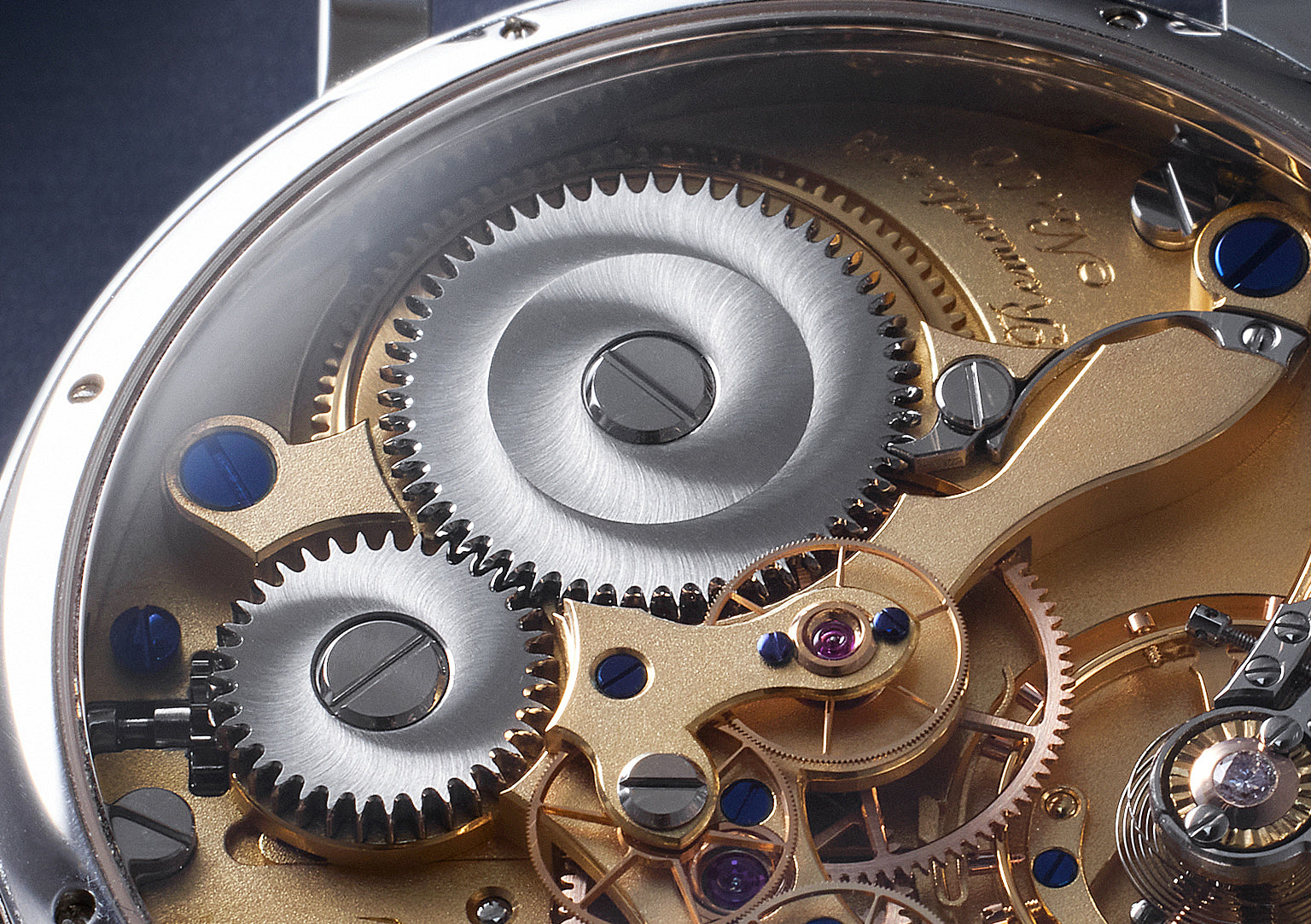The close-up image captures the intricate inner workings of a high-quality watch, showcasing an array of precisely crafted components. Dominating the upper center is a large, silver metal cog, with a smaller, interconnected gear just to its left. Both are meticulously enmeshed, demonstrating the precision engineering involved. The main body of the watch mechanism is primarily gold, highlighted by a rich array of gears and mechanical elements. Engraved into the gold in the upper right corner is a cursive script starting with a capital R and N, although the rest remains difficult to decipher. The image also spotlights several blue anodized screws securing the mechanism and a few embedded gemstones that add a touch of elegance. At the bottom center lies a distinctive copper-colored cog, and in the bottom right corner, a small wheel is partially visible, adjacent to a silver section of the watch's exterior casing. The upper right-hand corner features a navy blue background, contrasting with the watch's metallic hues. This detailed depiction likely represents the watch's underside, viewed through a glass back designed to showcase its craftsmanship.